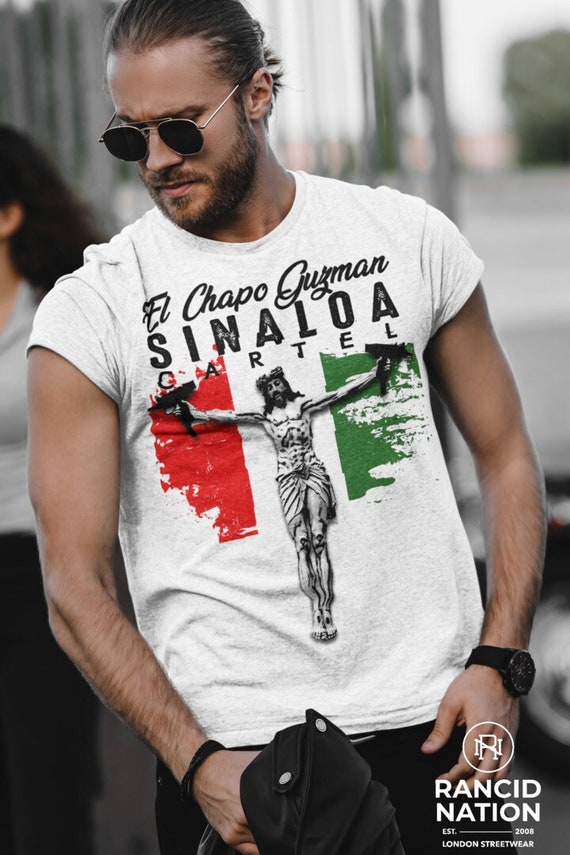The photograph depicts a man, possibly in his 30s or 40s, who bears a striking resemblance to a model. His medium brown hair is slicked back, and he sports dark sunglasses, a neatly trimmed mustache, and a beard. The man has tan skin and is wearing a white t-shirt emblazoned with the text "El Chapo Guzman Sinaloa Cartel." The t-shirt features an image resembling Jesus Christ in black and white, flanked by green and red elements on each side, symbolizing the Mexican flag. He has a black watch on his left wrist and holds a piece of clothing, possibly a jacket, in his right hand. The image includes additional details: in the bottom right corner, against a dark background, is the text "Rancid Nation Established 2008 London Street Wear." The man appears to be looking down towards the lower left corner of the picture. In the background, over his right shoulder, there is a woman in a white blouse and either black pants or a skirt, while over his left shoulder, the backdrop is mostly gray with a hint of green in the upper right corner.